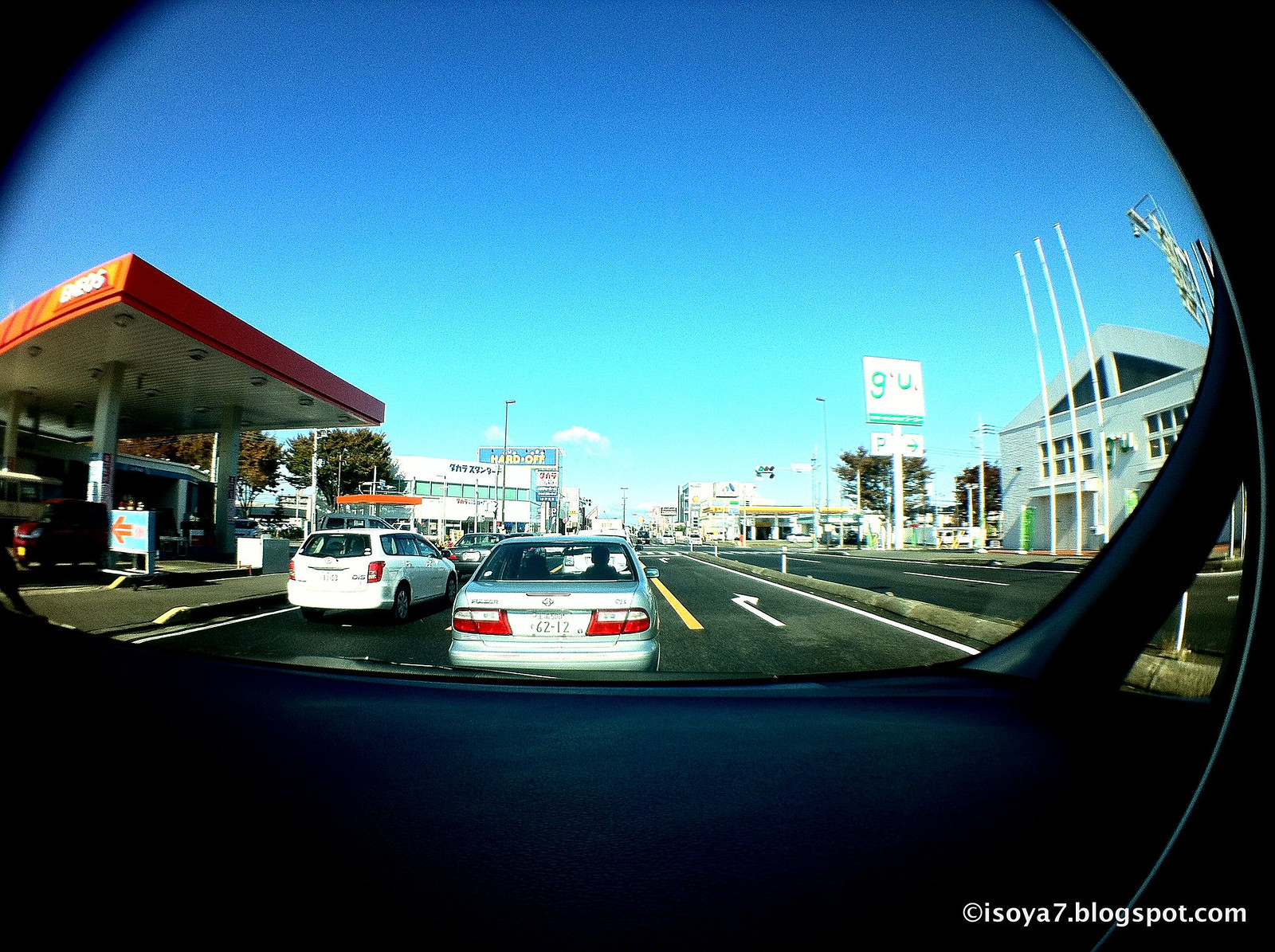This is a detailed photograph captured from a dash cam positioned on the passenger side of a moving vehicle, driving down a city street on a clear, sunny day. The image is credited to isoya7.blogspot.com, as noted in white text at the bottom right. The car is in the middle lane, with a white Toyota directly ahead. To the left of the Toyota, there is a smaller white car. The road has multiple lanes, separated by a curb—presumably dividing northbound and southbound traffic.

To the left of the street, there is a red gas station. On the right side, there is a store with a sign bearing green lettering on a white background that reads "GU." In the distance, buildings display Japanese lettering, indicating the photo was likely taken in Japan. Additional signage, including a "Hard Off" sign, is visible among the cityscape décor. The only interior details visible from the car are the dashboard and window frame. The photograph showcases a bustling urban environment with multiple vehicles and various business establishments on either side of the road.